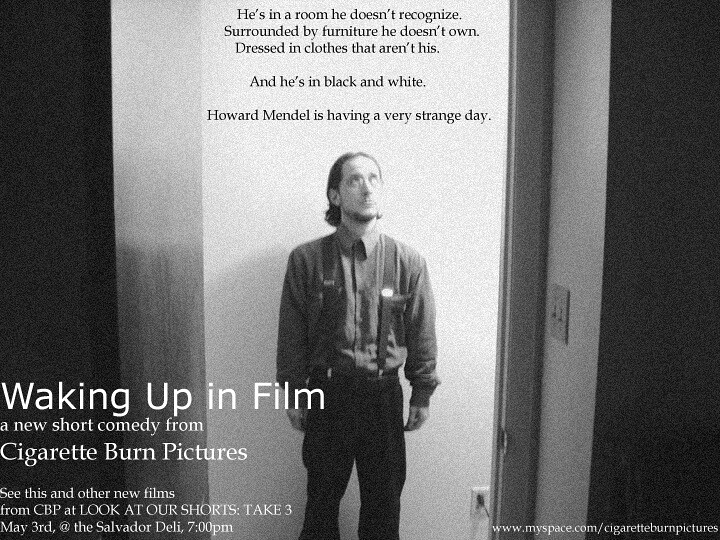The black and white image features a young man, Howard Mendel, standing directly at the center of an open doorway. He is looking upwards, clad in unfamiliar clothes—a buttoned shirt and black trousers. The room he finds himself in is also unfamiliar, filled with furniture that isn't his. The photograph captures him in a contemplative pose, his hair back-brushed and a beard accentuating his chin. The setting is indoors, with the room beyond the doorway appearing dark. To the right of the image, there is a light switch against a white wall. The image quality has a grainy, vintage feel, adding to the overall ambiance.

Text both above and below the image highlights the surreal nature of Howard's situation: "He is in a room he doesn’t recognize, surrounded by furniture he doesn’t own, dressed in clothes that aren’t his, and he is in black and white. Howard Mendel is having a very strange day." Additional text in the bottom left corner promotes the film: "Waking Up in Film, a new short comedy from Cigarette Burn Pictures. See this and other new films from CBP at 'Look at Our Shorts, Take 3,' May 3rd at The Salvador, Delhi, 7 pm." The website www.myspace.com/cigaretteburnpictures is also featured in the bottom right corner. This image bears the hallmarks of a film or play poster, effectively conveying its promotional message.